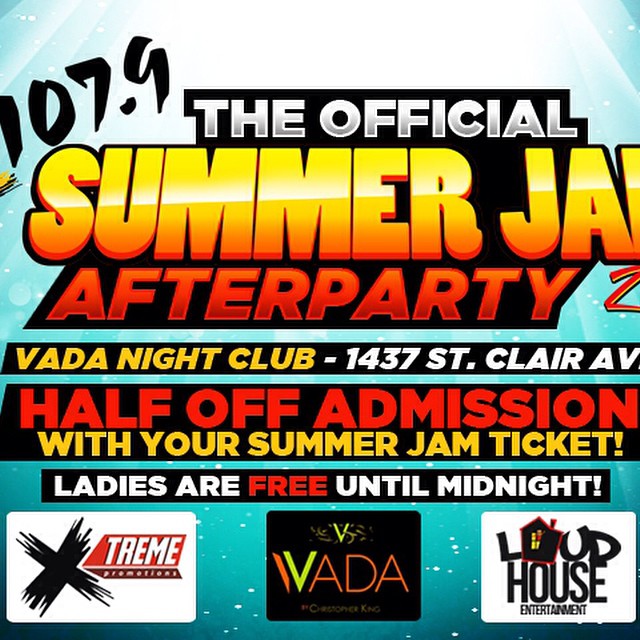This image is an advertisement poster for "107.9 The Official Summer Jam After Party 2" at Vada Nightclub, located at 1437 St. Clair Avenue. The poster’s background features a blue and white theme with some parts of the sign cut off on the sides. The text highlights that admission is half off with a Summer Jam ticket, and ladies get in free until midnight. At the bottom, there are three distinct squares featuring logos: the first square on the left has a black X with "X-treme" in red beside it; the middle square shows "V.A.D.A." in fluorescent green and brown lettering with a smaller neon V on top of a black square; and the third square on the bottom right displays the logo for Loud House Entertainment, with the "O" in "Loud" depicted as a black house with a red outline and a chimney.